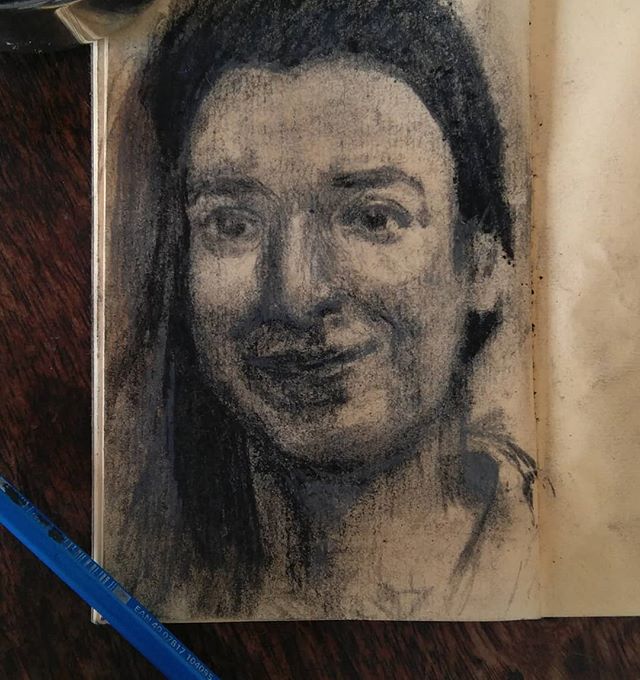This detailed charcoal sketch is displayed elegantly in a cherry wood frame, adding a touch of sophistication to the artwork. The sketch, rendered entirely in varying shades of black and gray, depicts a woman gazing forward with a contemplative expression. Her long hair cascades over her right shoulder, leaving her left ear visible and emphasizing the intricate details of her visage.

The artist has meticulously shaded her neck, creating a subtle depth that makes it appear slightly recessed. The woman's features are striking: her eyes are wide-set and piercing, framed by delicately drawn eyebrows. Her nose is broad, contributing to the expressive quality of her face. Her lips, partially shaded, add a sense of softness and realism to the portrait.

A notable element in the composition is a blue charcoal pencil, positioned diagonally across the bottom right corner of the frame, serving as both a tool and an accessory that hints at the creative process behind the artwork. The pop of blue contrasts vividly with the monochromatic palette of the sketch, adding an unexpected yet harmonious detail to the overall presentation.